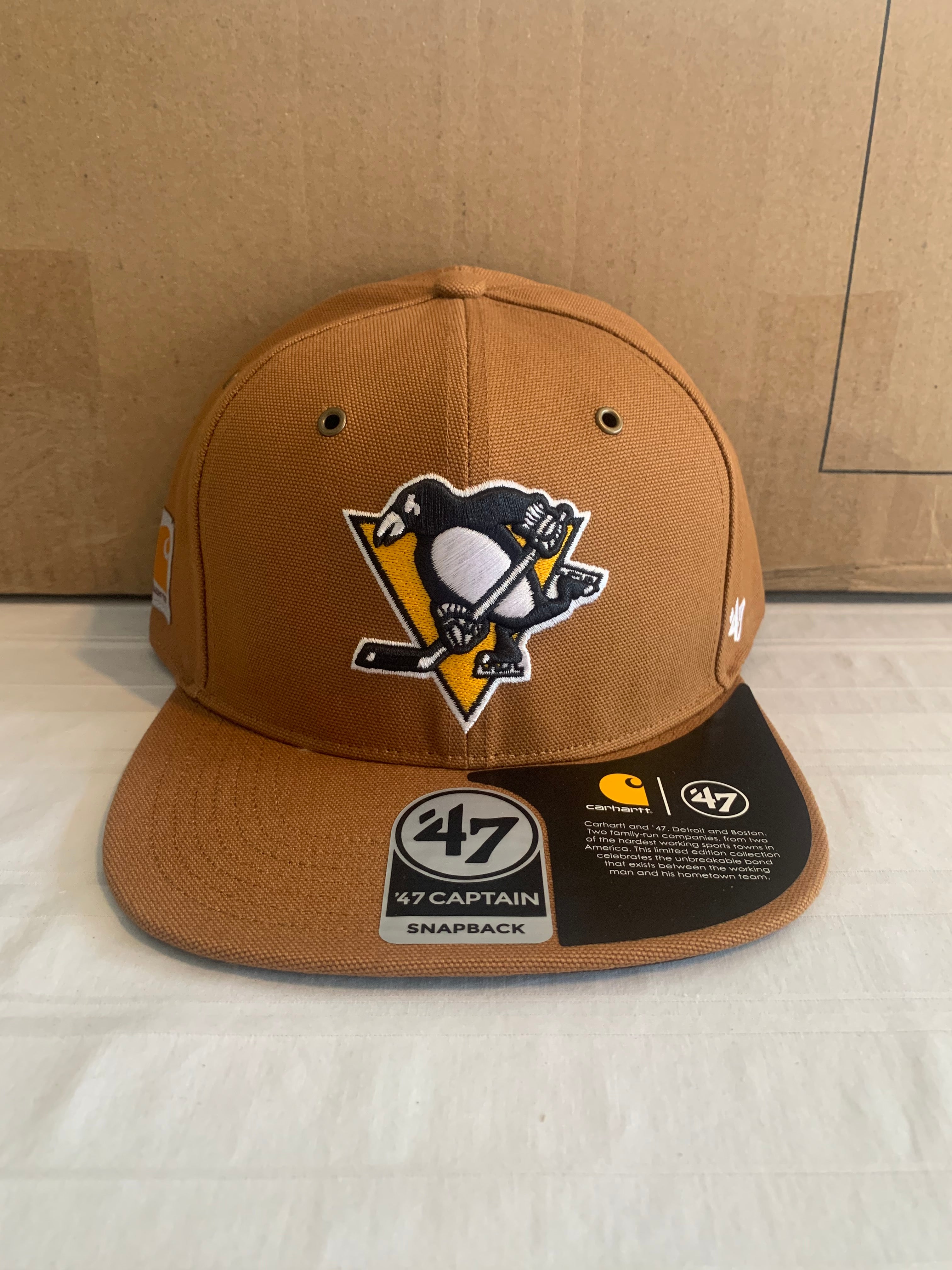In this vertically aligned rectangular image, we see a detailed depiction of a brown baseball cap with a flat brim, resting on a white tile floor. Behind the cap, there's a large cardboard box providing a tan background. The front of the cap features a prominent Pittsburgh Penguins logo, showcasing a black and white penguin holding a hockey stick against a yellow triangular backdrop. Attached to the brim of the cap is a black sticker with the brand label "47" and text indicating "snapback 47 captain." Additionally, there's a small circle with the number "47" inside it. The left side of the cap also carries a black label with intricate white text and a small yellow logo. This limited edition collection is a testament to the enduring bond between the working man and his hometown team, celebrating the collaboration between Carhartt and 47, two family-run companies from Detroit and Boston, renowned for their hardworking sports towns.